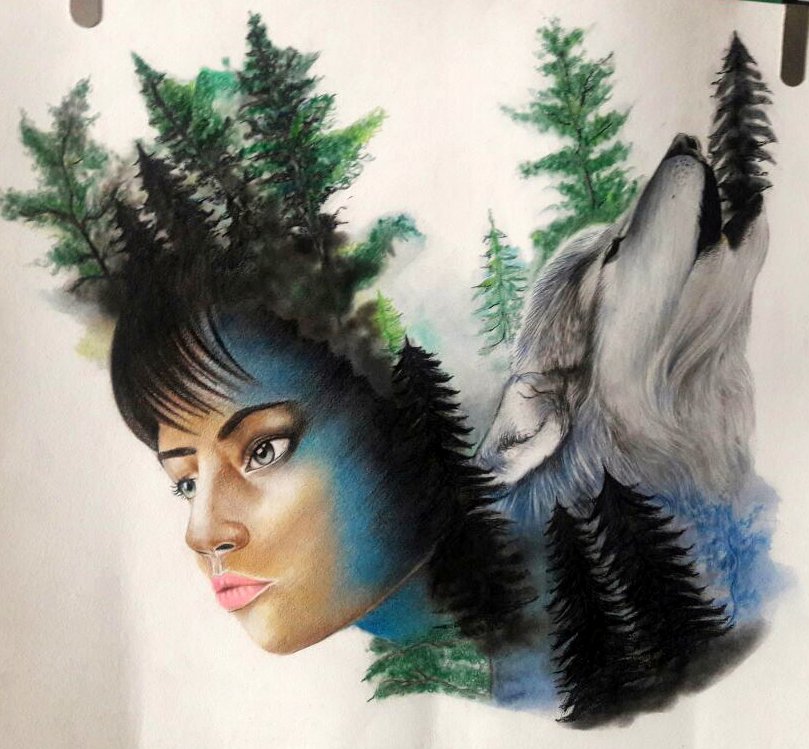This vibrant mixed media drawing, possibly created using pastels and colored pencils, features a compelling composition on white paper, clipped at the top with two silver clips. On the left side is a woman's face in a three-quarter angle, adorned with black bangs, pointy eyebrows, medium complexion, pink lips, and striking gray eyes. Her face transitions to a serene blue hue on one side, and from her hairline extends a forest of evergreen trees, blending into the scene as if sprouting from her head. On the right side of the image, a gray wolf with white lower fur and a black nose holds its head back in a dramatic howl. It has ears laid back, and its fur subtly tinged with blue, adding depth and contrast to its figure. The background behind the wolf is filled with both dark and green pine trees, unifying the natural elements with the woman's ethereal visage. The overall image seamlessly merges the human and natural world, creating a harmonious and detailed portrayal of coexistence.